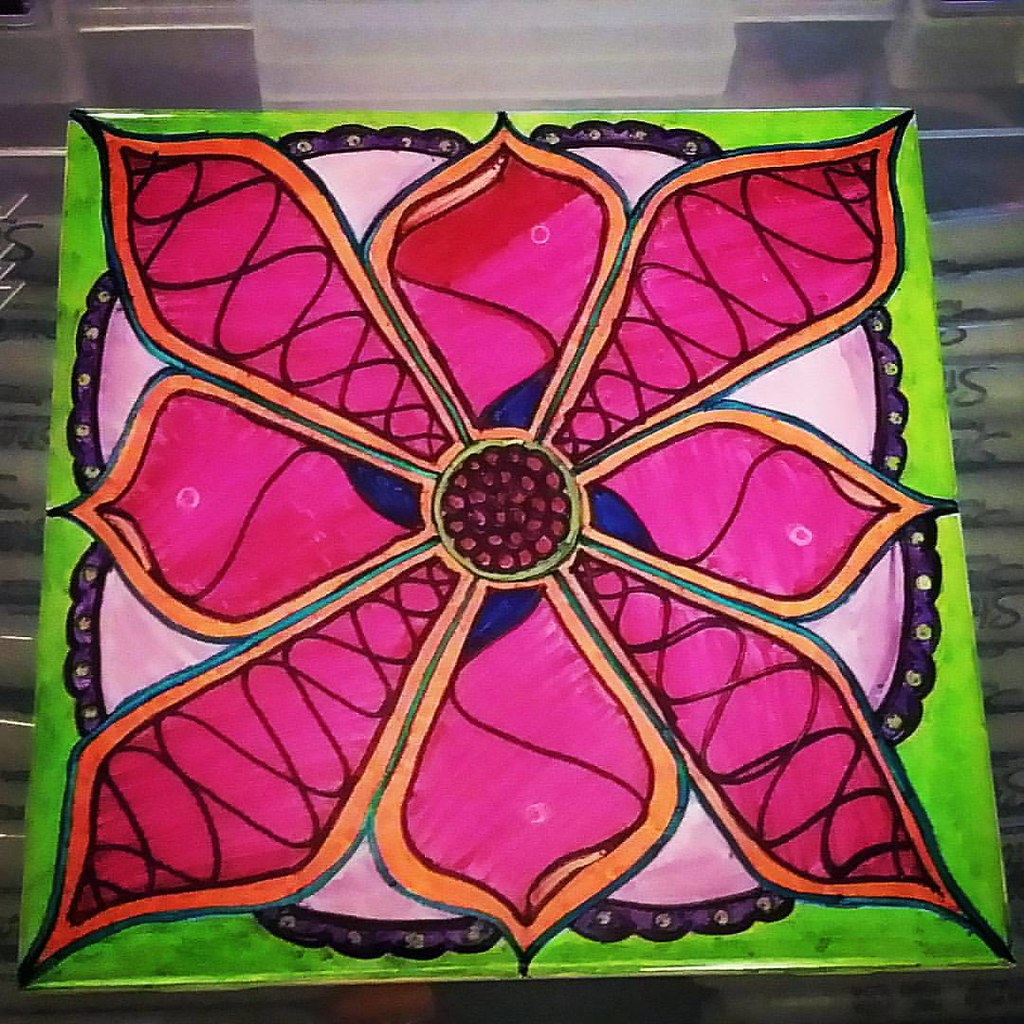The image features a brightly colored, glossy ceramic tile with a high-gloss finish that creates a reflective surface. At the center of the tile is a large, vibrant flower with deep magenta petals, each outlined in orange and teal, featuring a squiggly design running through them. The flower's circular center is adorned with small brown or burgundy dots, adding intricate detail. The background of the tile is a striking lime green, with a pink pillow-like element that has a purple scalloped trim edge. This pillow-like element includes yellow circles within the scallops. The tile is placed on an acrylic clear box, visible from an overhead perspective, which contains sharpie markers scattered inside. The overall composition of the image suggests an artistic project that has just been completed and is now being showcased.